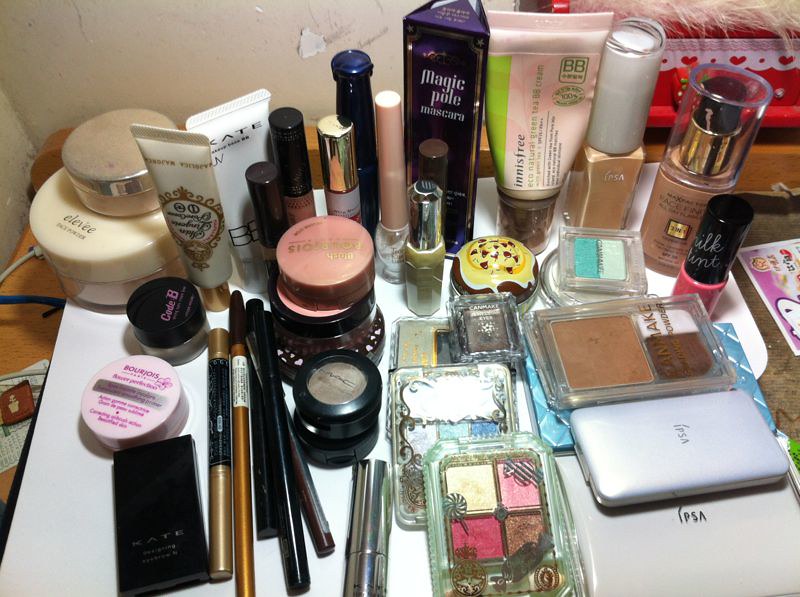This photograph captures an intricately cluttered vanity top, showcasing a plethora of beauty products. At the top of the image on one side, there are golden tan products accompanied by a variety of other items. Notably, there's a product with a black lid and pink font, a light pink product adorned with dark pink font, and a black container labeled "Engold" by Kate. Black and brown wands of makeup products are also prominent.

The assortment includes a white container of BB cream and various cover-up products with black lids. Among the notable brands, MAC products featuring black casings with tan powder stand out. Eye shadow palettes are scattered across the vanity, one featuring a vivid range of yellow, pink, dark pink, and brown shades. Another palette, designed with a desert theme, showcases colors reminiscent of cookies in shades of brown, yellow, white, and gold. Additionally, there are blue and light blue eye shadows visible.

A pink product with a black lid and a brown foundation bottle with a clear lid add to the mix. All of these products rest on a white surface. Nestled behind this array, a noticeable chunk of tan paint is missing from the wall, adding an imperfect yet realistic charm to the scene.